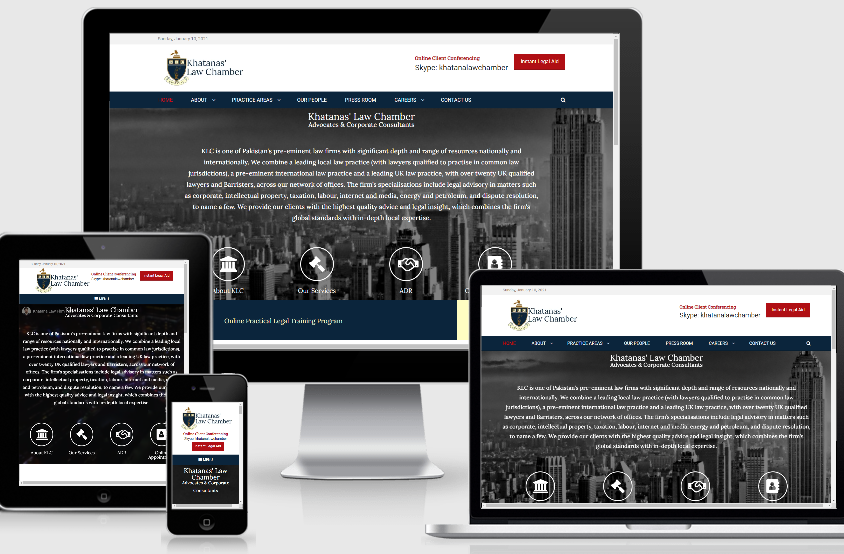This image is a screenshot of a webpage demonstrating its responsive design on multiple devices. In the background, there is a computer monitor on a stand displaying the webpage. In the foreground on the left, there is a tablet, resembling an iPad, and in front of it, an iPhone. On the right side at the bottom, a laptop is also showing the same webpage. The webpage appears to be for a law chamber, featuring a prominent white banner with a logo at the top, followed by a darker black banner with a menu. Below this, there's a photograph of buildings serving as a background for some descriptive text about the law chamber. Further down, there are icons and various options, culminating in a blue banner at the bottom. Despite slight variations in layout due to the different screen sizes, the content remains consistent across all four devices. The photograph is set against a very light gray background, emphasizing the devices.